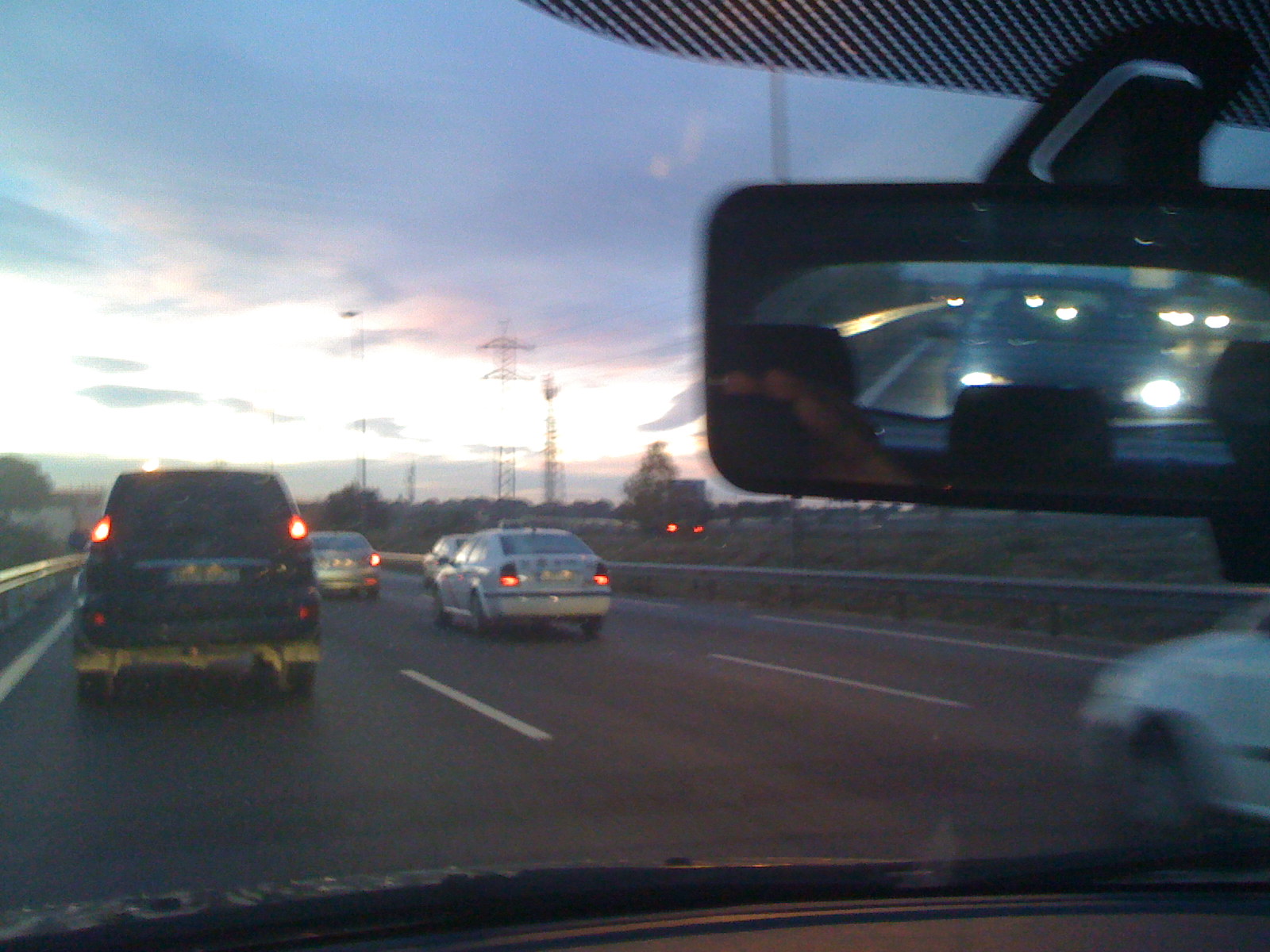A detailed and comprehensive caption for the image could be:

"Captured from inside a car with a smartphone, this photograph provides a viewpoint through the windshield from the driver's side. The picture includes the left side mirror and the rearview mirror, reflecting a car closely following with its headlights on. The rearview mirror also captures the reflection of the photographer's hand holding the phone. Ahead in the left lane is a blue SUV with its brake lights illuminated. In the middle lane, several vehicles with their lights on are visible. The background showcases a bright sky with scattered clouds, suggesting the onset of sunset as the day transitions into evening."